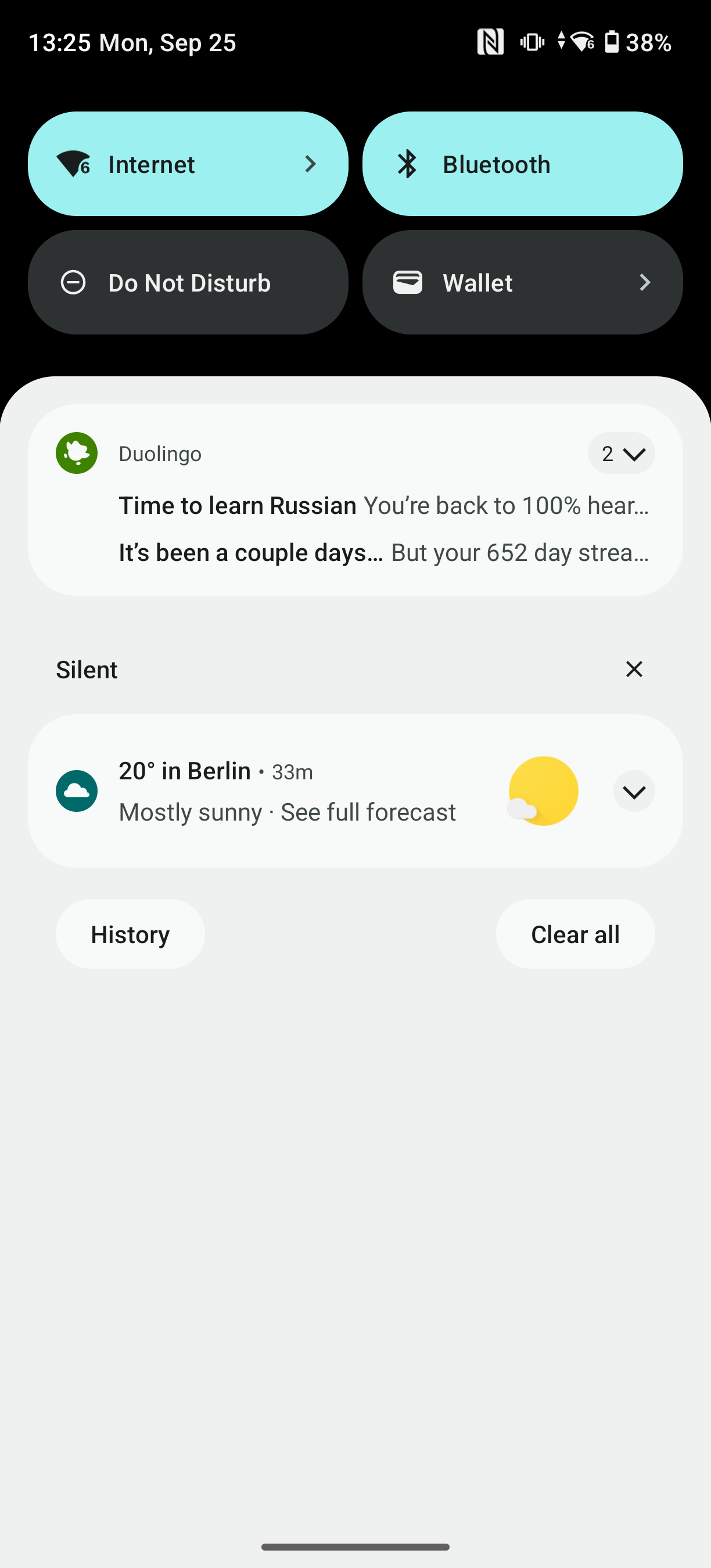A screenshot from a smartphone displays various notifications and system information. At the top of the screen, the clock shows 13:25 on a Monday in September. The battery icon labeled "SCP-25" indicates a 38% charge remaining. Symbols for Internet and Bluetooth appear within light blue ovals; the Internet icon resembles a downward-pointing triangle, and the Bluetooth symbol features a stylized "B" with split triangles on either side.

The status bar also includes icons for "Do Not Disturb" and "Wallet." The screen’s upper half has a black background, while the lower half transitions to gray. A notification from the Duolingo app reads: "Time to learn Russian! You’re back to 100% here... It's been a couple of days... but you're on a 652-day streak!" This message is followed by a "2" indicating another notification, and a "Silent" mode icon is present at the bottom of the screen.